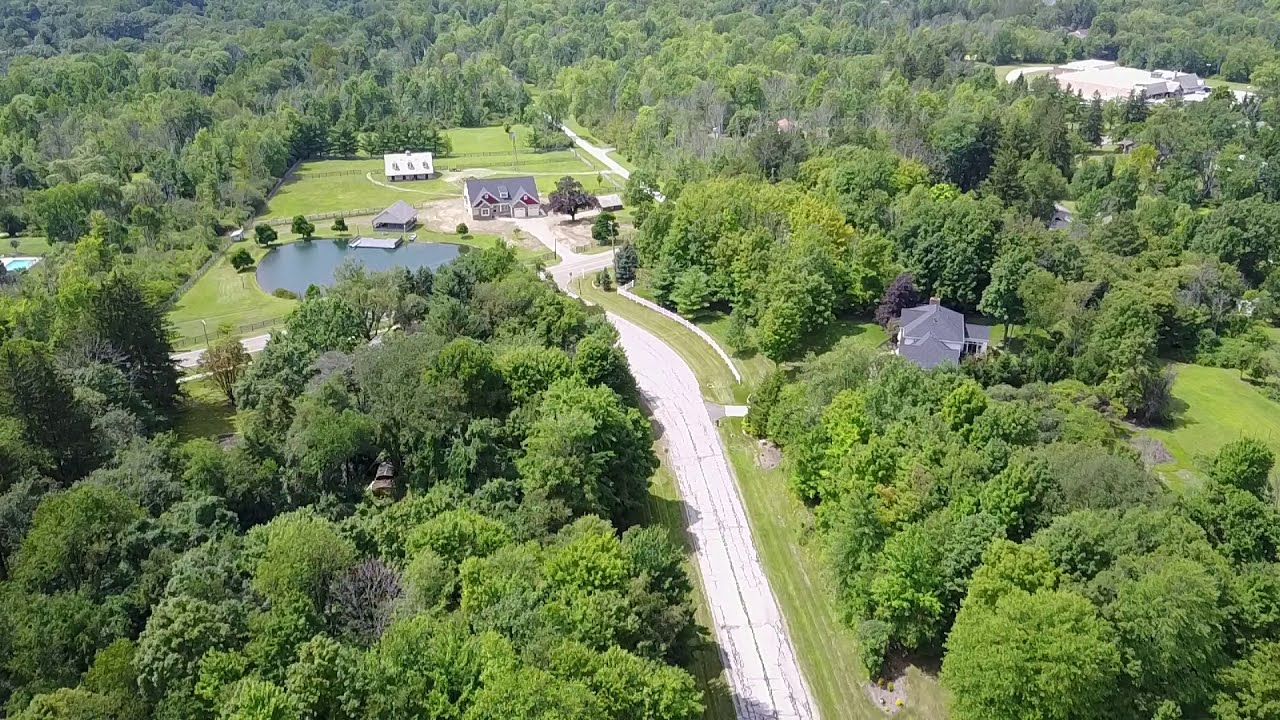This is an aerial photograph capturing a rural landscape. Dominating the scene is a verdant expanse with numerous green trees and patches of grass. The image features a narrow, white road running vertically through the center, providing access to scattered houses. The focal house, with two gables and a grey roof, is complemented by another house featuring a darker, purplish-blue roof off to the center-left. Adjacent to this house, a sizable pond is surrounded by grass and trees, with a pier extending into the water and a small structure on its edge. To the right, additional homes and sheds are visible amidst the dense foliage. The overall composition emphasizes the lush greenery and pastoral tranquility of the setting, under the clear daylight.